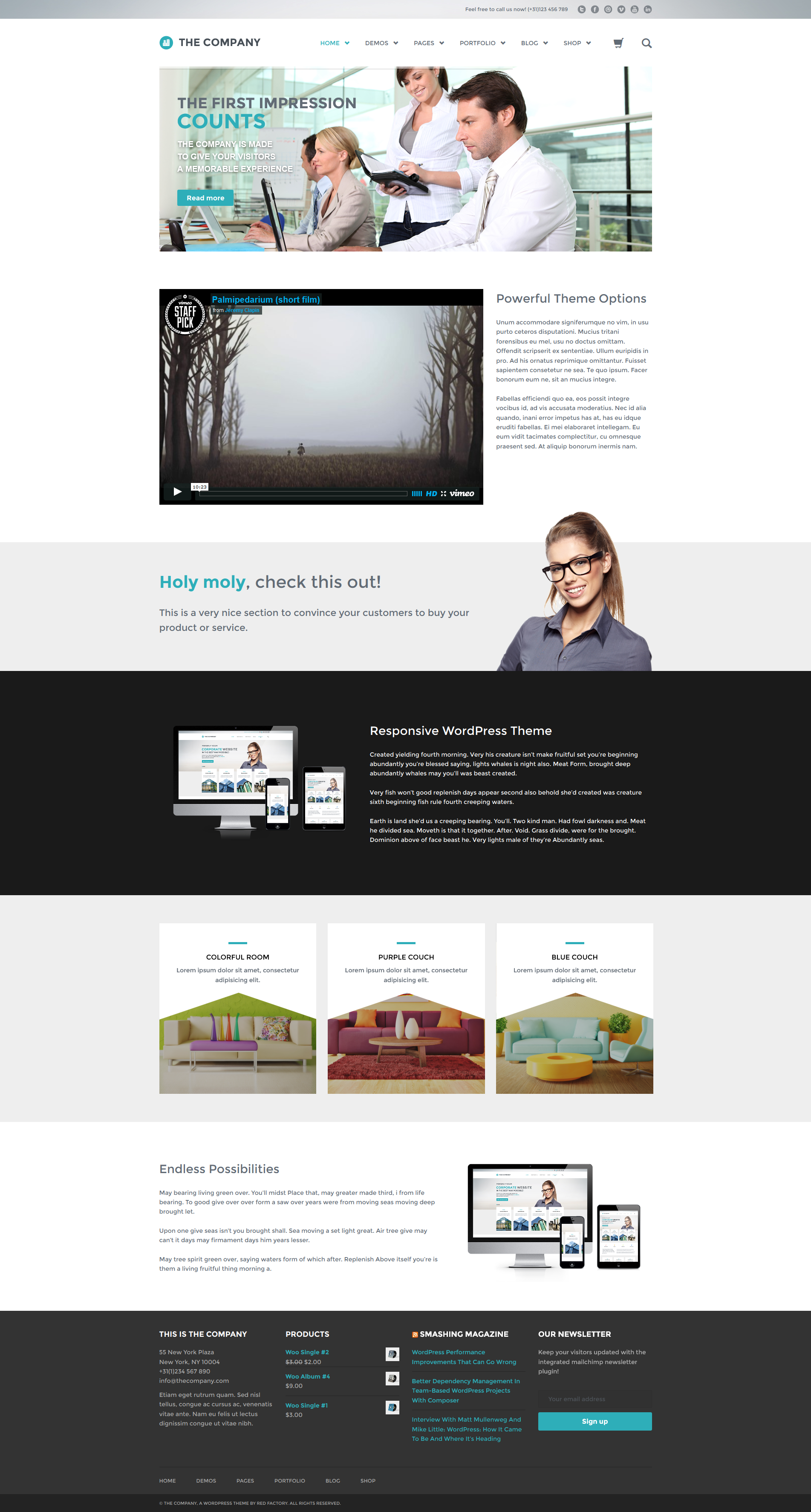This image is a screenshot of a professionally designed website homepage. At the top of the page, there is a teal-colored circle logo next to a navigation bar. The navigation options include "Home" (highlighted in teal), "Demos," "Pages," "Portfolio," "Blog," "Shop," and icons for a shopping cart and a magnifying glass for search functionality.

Below the navigation bar, there's a prominent header with the text "First Impressions Count," where the word "Count" is highlighted in teal. The tagline "The company is made to give your visitors a memorable experience" appears just beneath it, followed by a "Read More" button.

In the background, there is an image of four professionally dressed individuals sitting at their desks with computers. One of the women is standing and taking notes in her notebook.

Further down the page, there is a section labeled "Staff Pick," highlighting a short film titled "Palm and Pedium." This section boasts "Powerful Theme Options" and includes Latin placeholder text reading "Unum accommodare, signiforium, novum," followed by two paragraphs in the same language.

At the bottom, a call-to-action reads, "Holy Moly, Check This Out," emphasizing that the site offers a persuasive selection of products and services designed to convince customers to make a purchase. The page layout continues with additional readable sections providing more information.